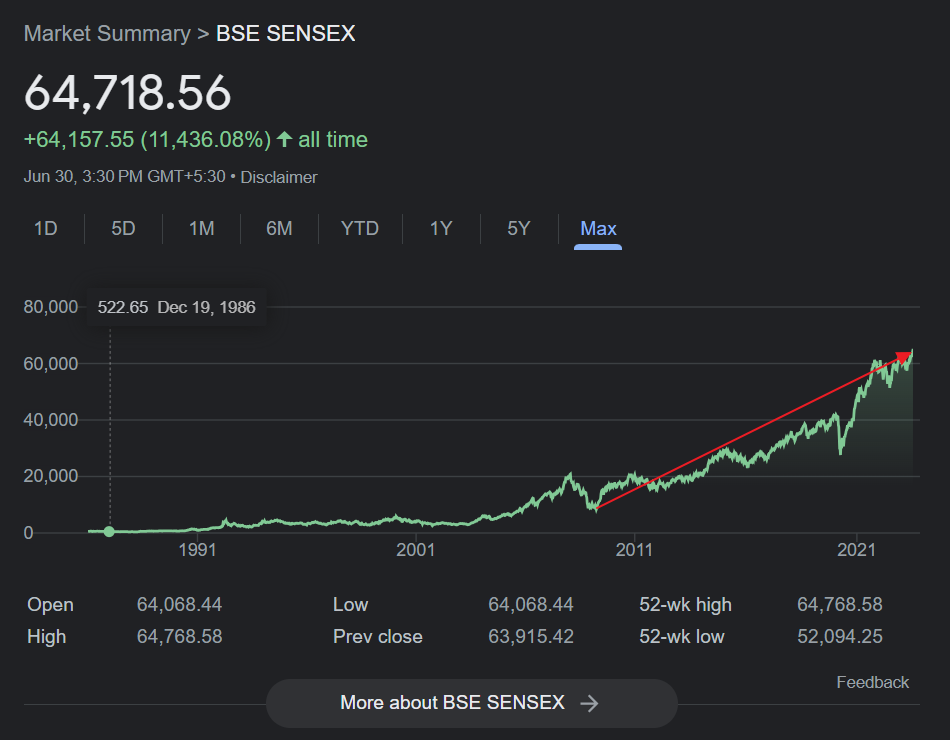This image showcases a detailed market summary for the BSE Sensex. At the top, the bold heading reads "Market Summary: BSE Sensex." Just below this heading is the current value of the index, marked at $64,718.56. Displayed prominently in green, the index is noted to have risen by $64,157.55. Additionally, it indicates an all-time increase of $11,436.08.

Further down, the image shows the specific time and date of this summary. Beneath this time stamp are several clickable small squares allowing viewers to analyze the market trend over different periods: 1 day, 5 days, 1 month, 6 months, Year to Date (YTD), 1 year, 5 years, and Max. The "Max" option is currently selected and highlighted in blue.

Below these time-range selections, a line graph is presented to visually represent the market trends. The graph includes a prominent green line, indicating the trajectory of the stock, and a red arrow edited onto the photo pointing from 2011 to 2021, signifying a specific period of interest.

At the bottom of the image, key market details are listed: Open, High, Low, Previous Close, 52 Week High, and 52 Week Low. This detailed presentation provides an insightful overview of the BSE Sensex market summary.